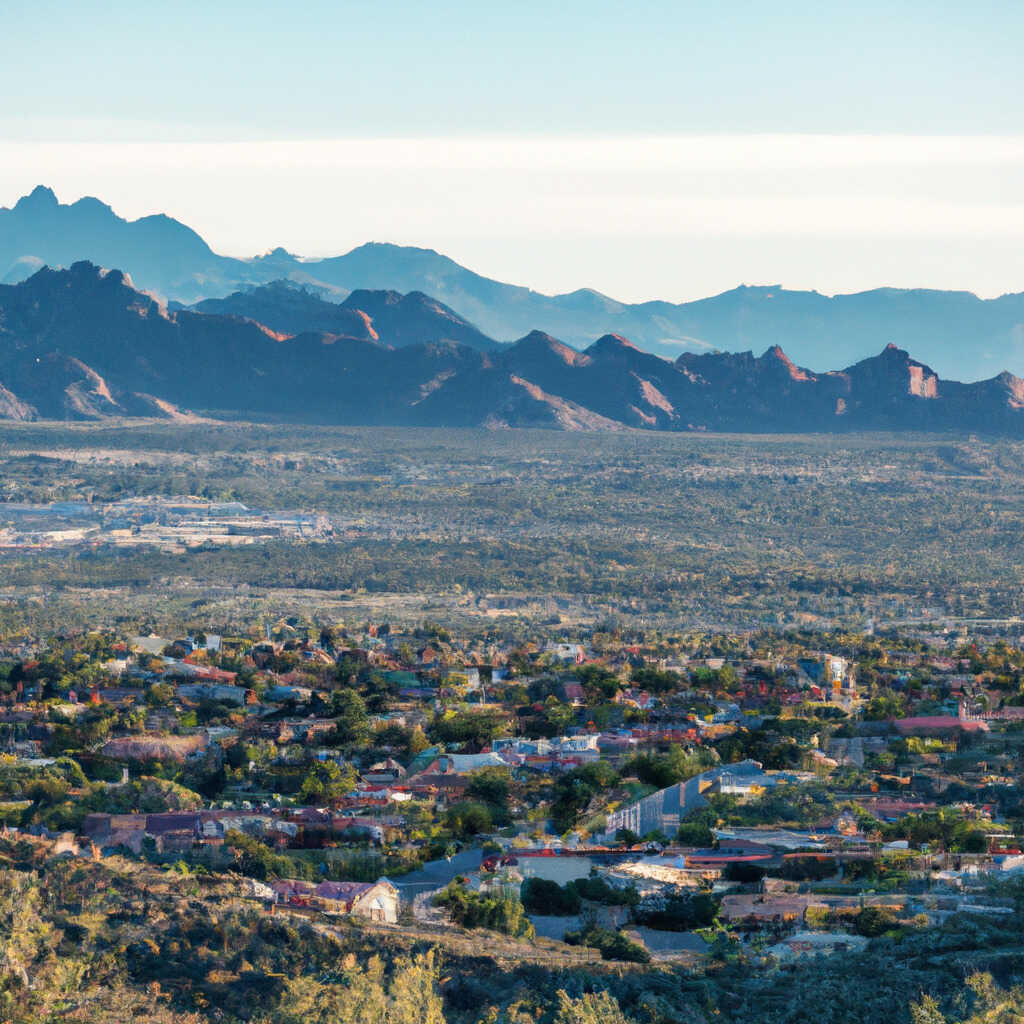This panoramic aerial shot captures a large, sun-baked valley framed by a majestic, multi-layered mountain range in the background. The sky is a hazy blue-white, providing a serene canopy over the scene. The mountains stretch across the entire width of the photo, with one set of hazy peaks seeming almost like a reflection due to the atmospheric conditions. In the foreground, a lush neighborhood with numerous houses, roads, and verdant trees is vividly visible, extending toward the middle of the image. Beyond this urban area, the landscape transitions into barren plains with sporadic greenery, indicative of a more rural setting. Nested amidst this plains area are patches of white fencing enclosing green vegetation, adding a structured appearance to the otherwise rugged terrain. The overall scene beautifully encapsulates the contrast between developed neighborhoods and untouched natural plains, all under the watchful presence of the distant mountains.